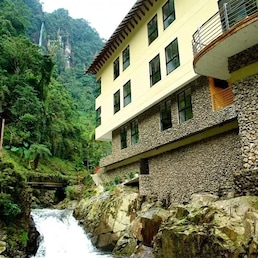This photograph captures a detailed view of a large, four-story house situated near the shore of a rushing river. The house is divided into two distinct sections: the top part is painted a light yellow and includes multiple windows, with eight windows visible in total. Additionally, there's a balcony with a gate and sliding doors in the upper right-hand corner. The lower part of the building is constructed from brownish-gray stone, blending seamlessly with the surrounding rocky terrain. Below the building, a river runs vigorously over the rocks. To the left of the building, the scene is framed by lush, dark green trees and bushes, which continue into the background and start to blur as they recede into the distance. In the far upper right corner of the image, another structure can be seen partially obscured by the dense foliage.